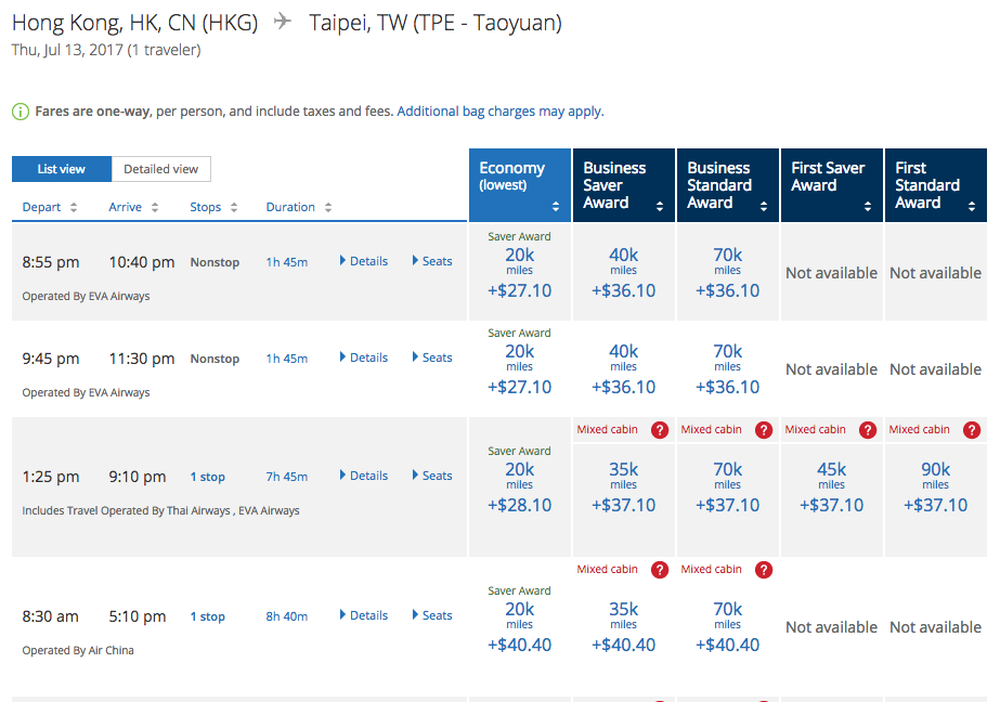The image features a white background with black text at the top. It reads: "I'm Hong Kong, HK, CN (HKG)" followed by an airplane icon and the text: "Taipei TW (TPE) - Taiwan." Beneath this, the date is specified as Thursday, July 13th, 2017, with a note that it pertains to "one traveler."

Further down, a disclaimer states: "Fares are one way per person and include taxes and fees. Additional bag charges may apply." 

Below this disclaimer, there are two buttons: a dark blue button on the left labeled "List View," and a white button on the right labeled "Detailed View."

Under the buttons, there is a table with four columns titled: Depart, Arrive, Stops, and Duration. To the right of these columns, there are five additional columns titled: Economy Lowest, Business Saver Award, Business Standard Award, First Saver Award, and First Standard Award.